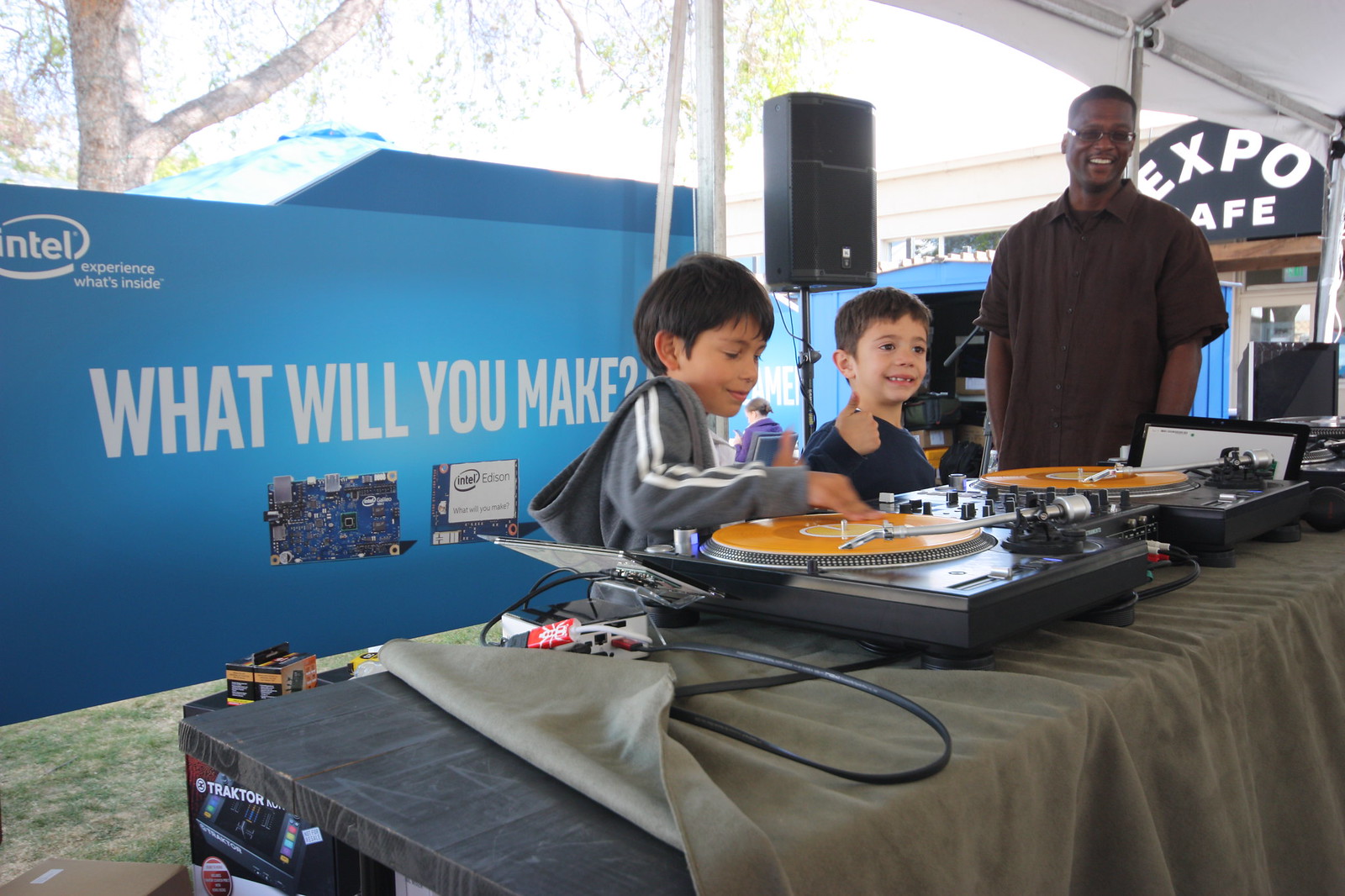In this engaging photo taken at an outdoor event, likely an expo or family farm market, three individuals—a man and two young boys—are gathered around a DJ station covered with an olive green tablecloth. The two boys, each with dark hair, are actively engaging with the DJ equipment, which includes what appear to be record players and other sound equipment with visible cords. The first boy, wearing a gray hooded sweatshirt, focuses intently on the equipment, while the second boy, dressed in a black shirt, beams directly at the camera. The adult, a black man with glasses adorned in a short-sleeved button-down brown shirt, stands to the right of the boys, smiling warmly at their enthusiasm. Behind them, a blue banner prominently displays the Intel logo and the slogans "Experience What's Inside" and "What Will You Make?" in large white letters, accompanied by images of microchips. An upright speaker is positioned to the left of the man, further setting the scene of an interactive and educational display.